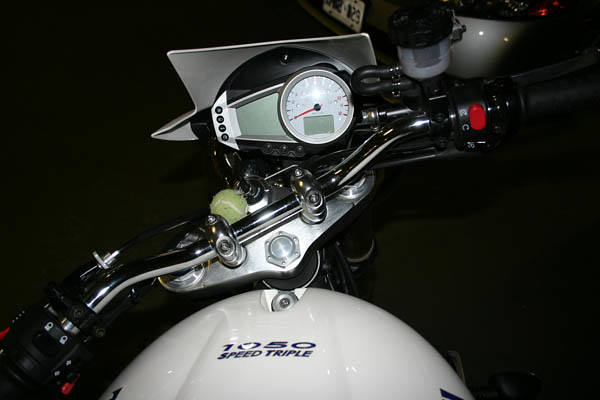The image is a close-up shot of the handlebars of a motorcycle, adorned with various gauges and devices. The handlebars are equipped with multiple knobs and buttons designed for manipulation while riding. Prominently, there is a key with a tennis ball keychain attached, inserted into the ignition. Mounted atop the center of the handlebars are cumbersome-looking gauges, including a speedometer and other instruments that are not immediately identifiable. The motorcycle’s body is partially visible and is white, with the model name "1050 Speed Triple" displayed in blue text. The background appears completely black, suggesting the photo was taken at night, though faint outlines of a license plate and potentially some taillights are discernible. The additional devices mounted on the handlebars are arranged in such a way that they look like they could obstruct the rider's vision.